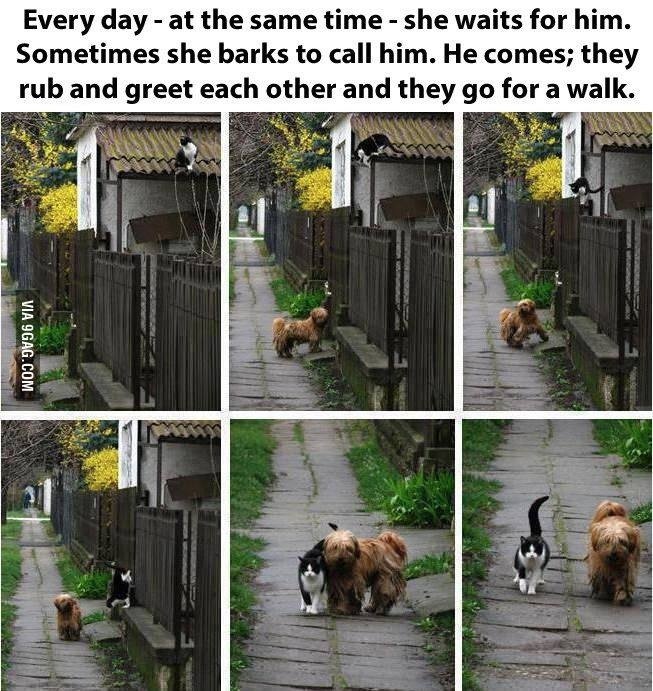The graphic features a series of six photographs that chronicle the daily routine of a small brown shaggy dog and a black and white cat. At the top of the graphic, black text reads: "Every day, at the same time, she waits for him. Sometimes she barks to call him. He comes, they rub and greet each other, and they go for a walk."

In the first photo, the dog is seen waiting by a fence as the cat perches on a roof above. The second photo captures the cat beginning its descent onto the fence where the dog eagerly waits. As the cat lands on the fence in the third photo, the dog takes a step back in anticipation. The fourth photo shows the cat making its final jump from the fence to the sidewalk. In the fifth photo, the cat affectionately rubs against the dog, greeting it warmly. Finally, in the sixth photo, the inseparable duo strolls down the sidewalk together, showcasing their unique bond and daily companionship.